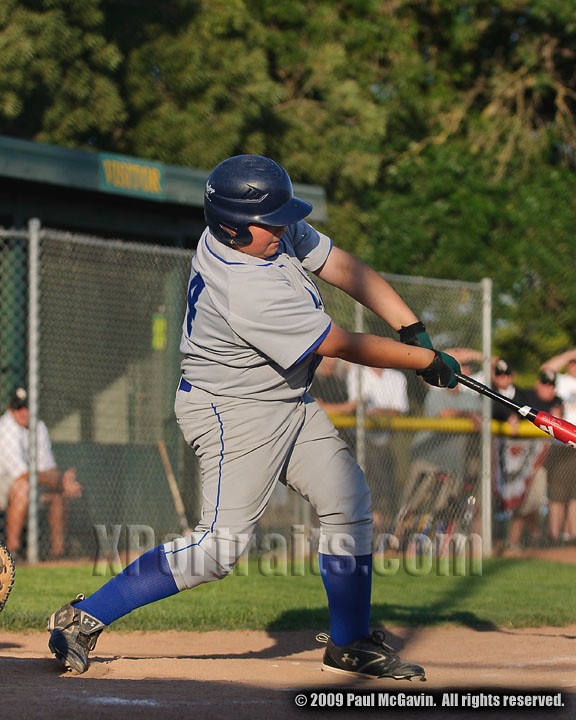The photograph captures an action-packed, late evening Little League baseball game. Centered in the image is a slightly pudgy, young Caucasian boy, dressed in a predominantly gray uniform with blue accents. He’s mid-swing at home plate, gripping a black and red bat while wearing green batting gloves and a dark blue helmet. His blue tube socks complement his well-worn black Under Armour cleats, with the logo prominently visible on one shoe. The player's figure is mostly in profile, facing right, against the backdrop of a chain-link fence. In the out-of-focus background, to the left, a seated adult in a white shirt and black hat is visible, while on the right, other spectators casually lean against a yellow barrier. The scene is suffused with the warm, orange light of the setting sun, highlighting the boy's concentrated effort. The image, which hints at the boy just making contact with the ball, bears an embossed watermark near the bottom that reads "xportraits.com" and a black bubble in the bottom right corner stating "Copyright 2009, Paul McGavin. All rights reserved."